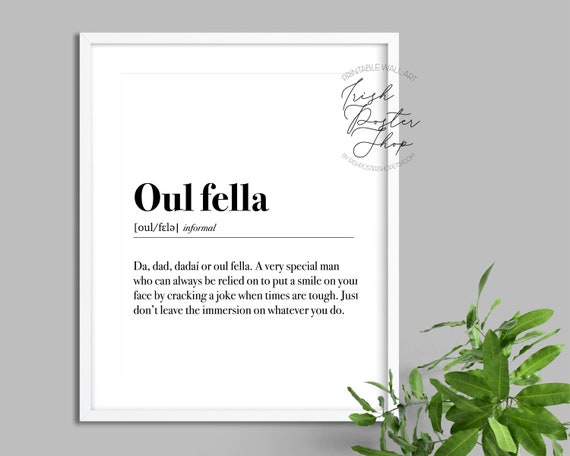The image showcases a gray wall adorned with a framed art print in the center. The art print features a thin white border and central text that reads in black, "OULFELLA," with a pronunciation guide below it and the word "informal" beneath a horizontal black line. The descriptive text says: "Da, Dad, Da Day, or Owlfella, a very special man who can always be relied on to put a smile on your face by cracking a joke when times are tough. Just don't leave the immersion on whatever you do." At the upper right of the frame, there is a watermark in script, partially readable, indicating it is from a poster shop. In the bottom right of the image, a green potted plant adds a touch of nature to the scene. The wall color is consistent with all descriptions, being light gray or blue-gray.